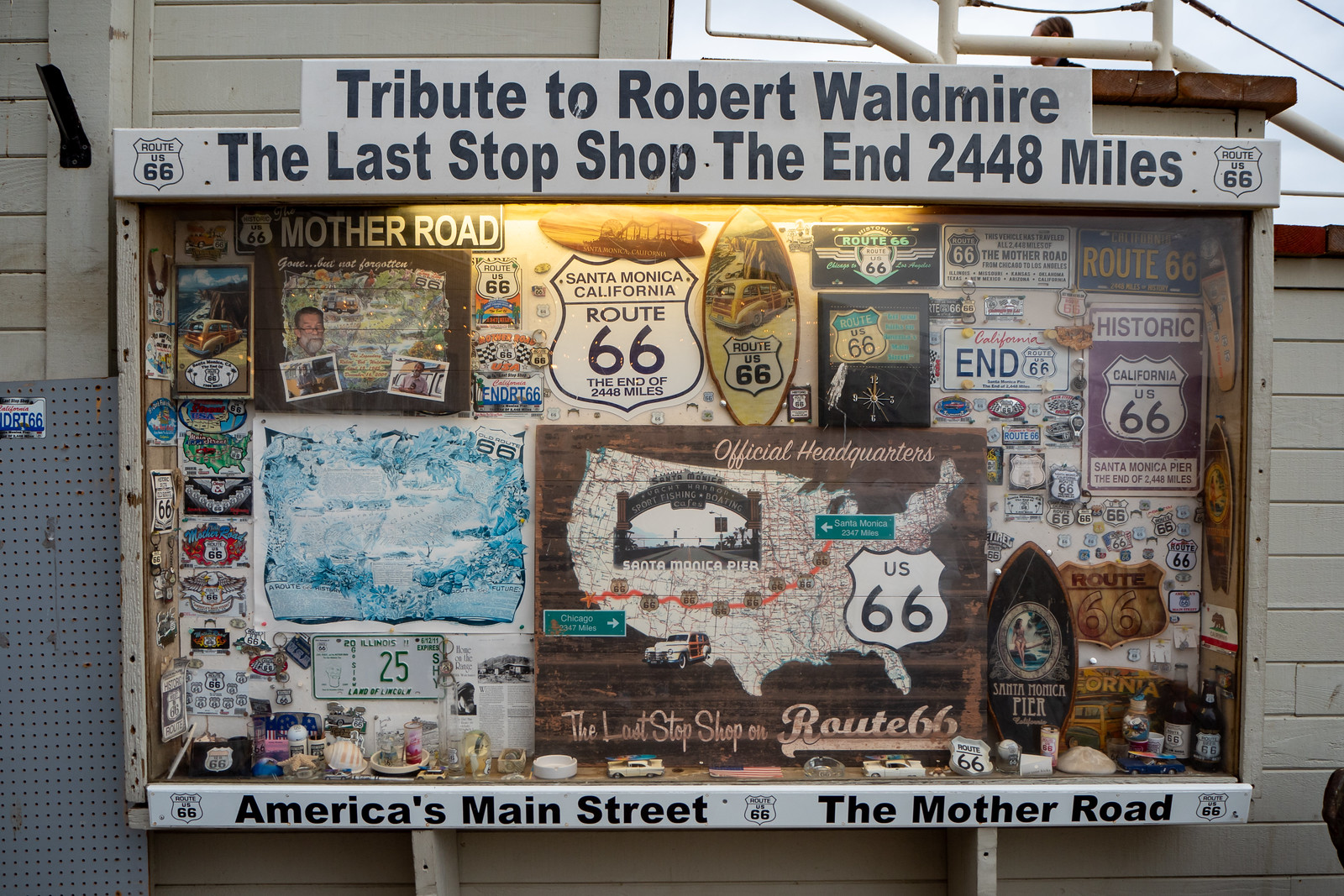The image depicts a detailed diorama dedicated to Route 66, prominently featuring a tribute to Robert Waldmeier. This tribute, set against the outside wall of a building, encased in a distinctive white metal box with wooden side frames, displays an intricate collection of Route 66 memorabilia. The building wall behind it is constructed of plain tan plank walls with a dark gray metal sheet on the left side, which features a license plate and a hose.

The diorama's main board begins at the top with blue text stating, "Tribute to Robert Waldmeier, the last stop shop, the end, 2,448 miles," flanked by Route 66 logos. Below, various items narrate the history and charm of Route 66: maps of the United States highlighting the route, whimsical models of cars, license plates, ashtrays, shells, photographs, and even a miniature surfboard. This comprehensive collection showcases stops along Route 66, featuring an orange line depicting the route and significant landmarks like the Santa Monica Pier.

Smaller captions and tags include phrases like "America's Main Street," "the mother road," and "Gone but not forgotten," signifying the nostalgic and historic essence of the famous highway. The vibrant display is colorfully adorned with red, blue, brown, yellow, purple, black, and white, reflecting the diverse memorabilia and the vibrant legacy of Route 66.